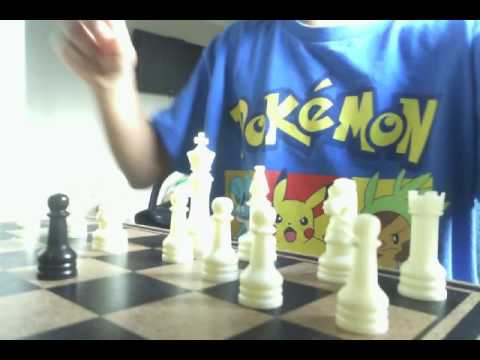The image portrays a scene of a young boy playing chess, captured at an approximate 30-degree angle. The focal point is the chessboard, composed of a gray or off-white and black checker pattern, predominantly showing white pieces with only one visible black pawn to the left. The board is flanked by black bars at the top and bottom, suggesting it might have been taken from an older, grainier video.

The young boy, identifiable by his right arm and bright blue Pokémon T-shirt, sits behind the white pieces, ready to make a move. His shirt features the word "Pokémon" in yellow letters above images of several Pokémon characters, including Pikachu in a red box, and possibly Squirtle in a yellow box, though some characters are partially obscured by the chess pieces.

In the background, a white wall is visible with a black flat-screen TV mounted on it. Light streaming through a window oversaturates the left side of the image, adding a bright glow that partially obscures some of the white chess pieces and further accentuates the scene's nostalgic, vintage feel.